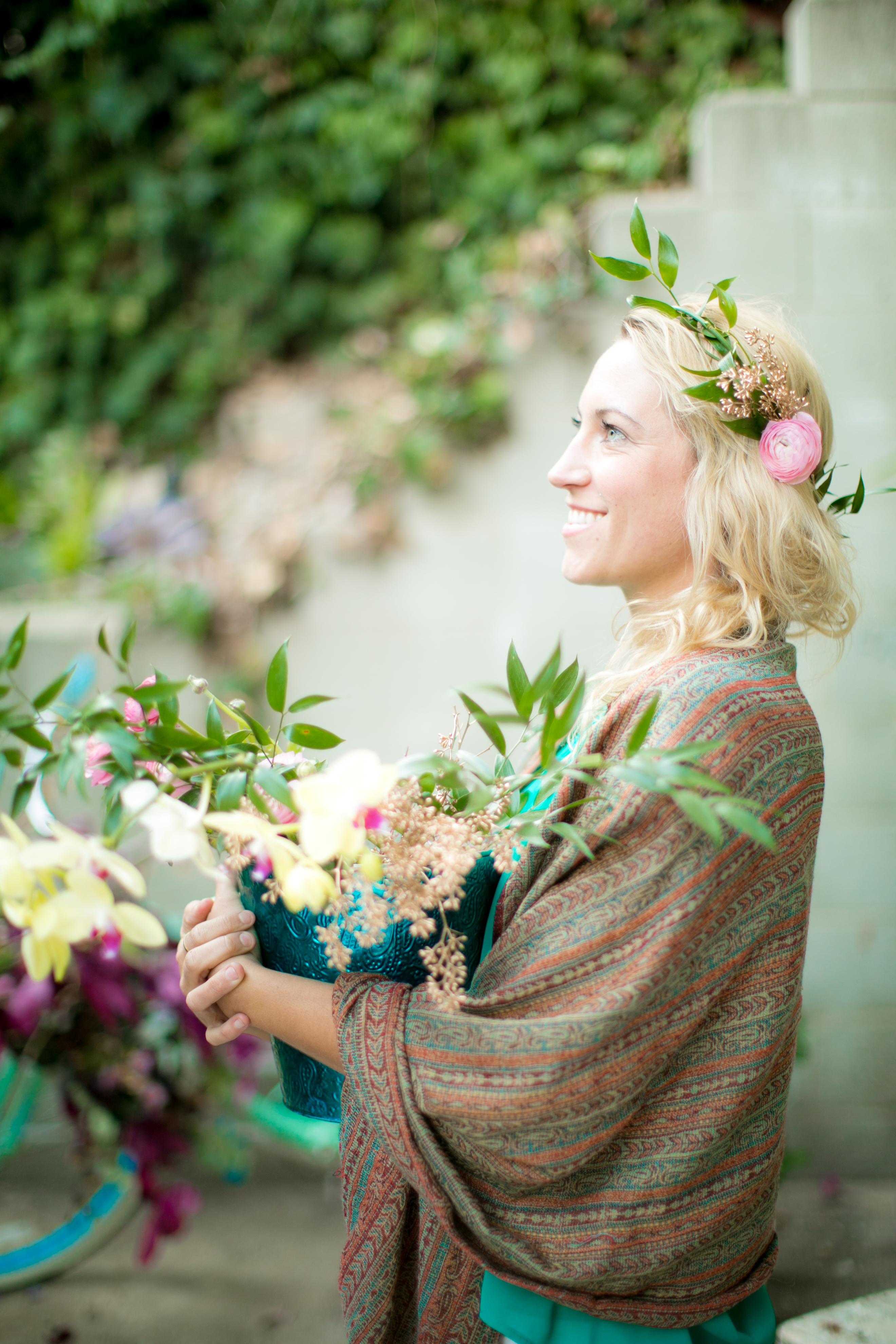A smiling woman with fair skin and blue eyes is gazing slightly upwards to the left. She has shoulder-length, slightly wavy blonde hair adorned with a green headband made of leaves and flowers, including a prominent pink flower over her ear, as well as smaller pink and white flowers. She wears light makeup and a turquoise blouse or dress, partly covered by a tan and orange shawl with hints of turquoise. She's holding a dark teal bucket filled with flowers that mirror the ones in her hair—light yellow orchids with red centers, various green leaves, and some pink, small peach-colored flowers. Behind her is a brick retaining wall with foliage, and in the background, there's a blurred image of a turquoise bicycle and some trees.